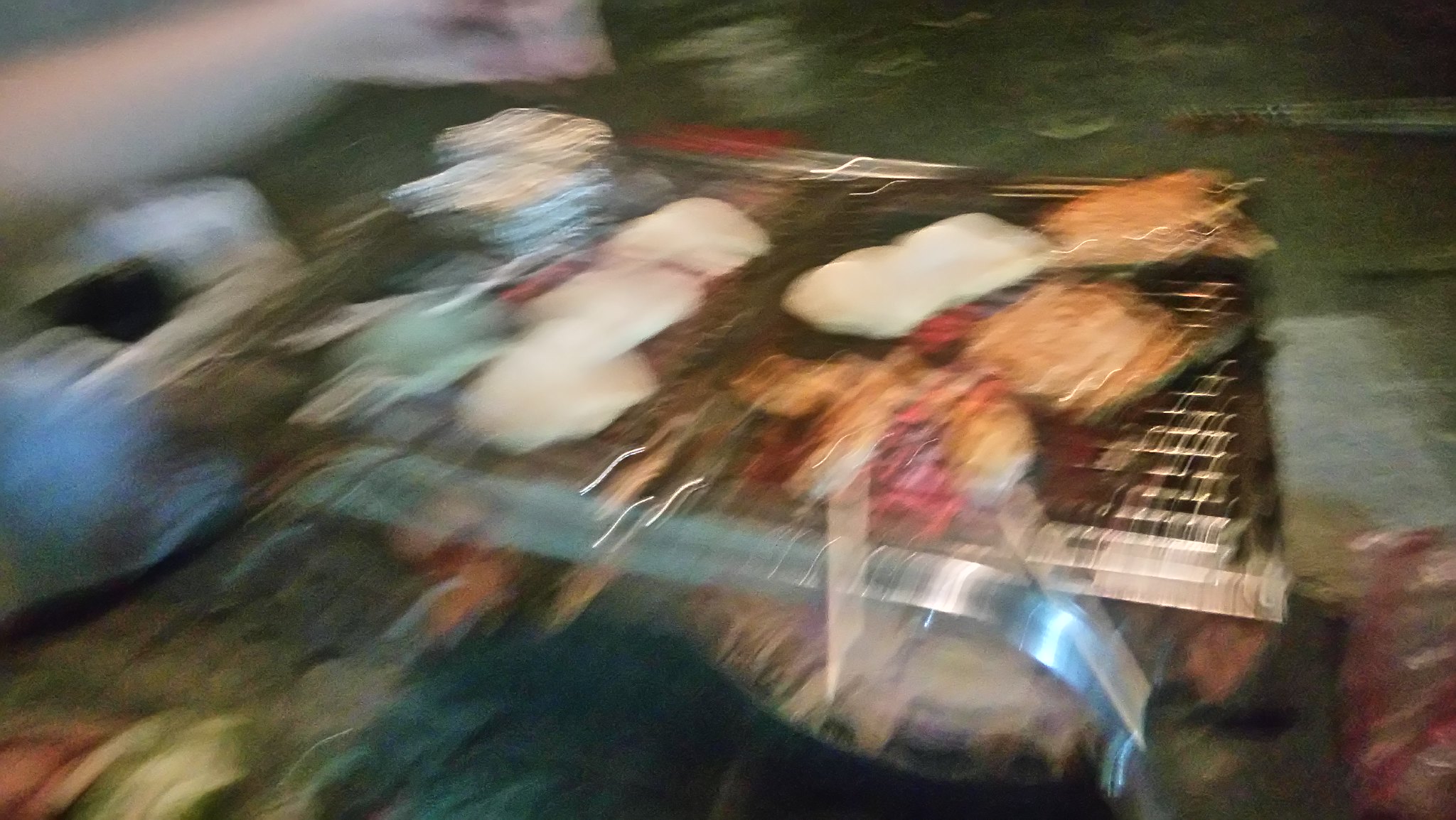The blurry image depicts the top view of what appears to be a grill. Though the image quality makes it challenging to discern details, the setup suggests an outdoor cooking scene. A heat source, likely flames, is visible coming from below, indicating that the grill is in use. The grilling surface features a handle that extends outwards, possibly serving as support or a foot for the grill. On top of the grill, there are three slices of steak situated towards the right-hand side. Additionally, a piece of tinfoil can be seen on the upper left corner of the grill surface, hinting at ongoing food preparation.